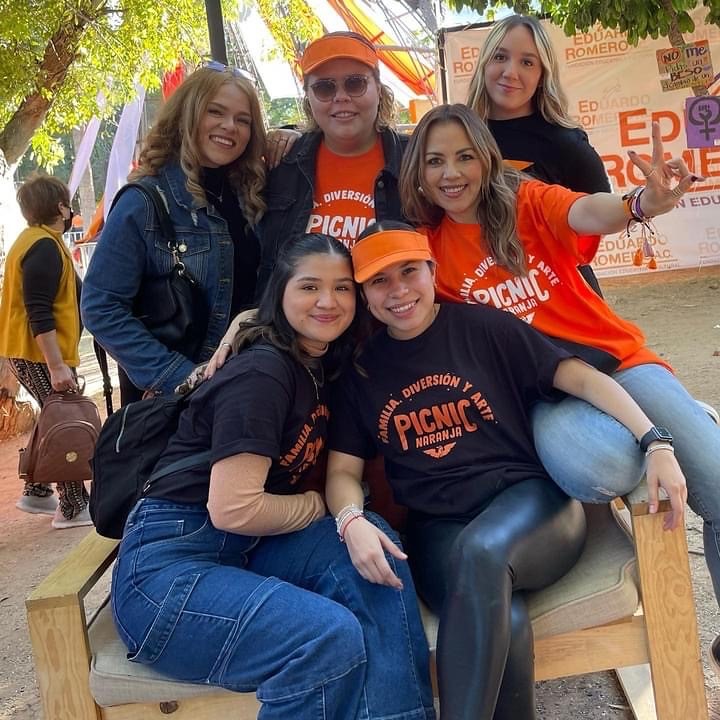In this vibrant, sunlit photograph, a group of six young Hispanic women, all appearing to be in their twenties to thirties, are gathered at an outdoor event, likely a family reunion titled "Familia Diversión y Arte Picnic Naranja." They are seated on an oversized, wooden chair, posing closely together while smiling at the camera. Their attire is a mix of event-themed shirts—some in orange with white lettering, and others in black with orange lettering. Two women sport orange visors, adding a splash of color to the group. One of the women in a black T-shirt and gray spandex pants has her left arm resting on the chair's arm, covered in bracelets and a watch, while another woman showcases a peace sign with her left hand. 

The lively setting features bright green leaves on nearby trees, indicating a sunny day. Compact dirt covers the ground, and various banners and signage, including a prominent "Edward Romero" sign, decorate the background. Adding to the scene’s detail, a woman in a jean jacket with a black purse is situated on the left of the group, and another in a dark jacket and sunglasses stands out on the right. In the backdrop, an older woman, possibly in her sixties, walks by with a backpack and a face mask, clad in a yellow vest, hinting at ongoing activities. Altogether, this image captures a joyful moment of unity and celebration at this outdoor picnic event.